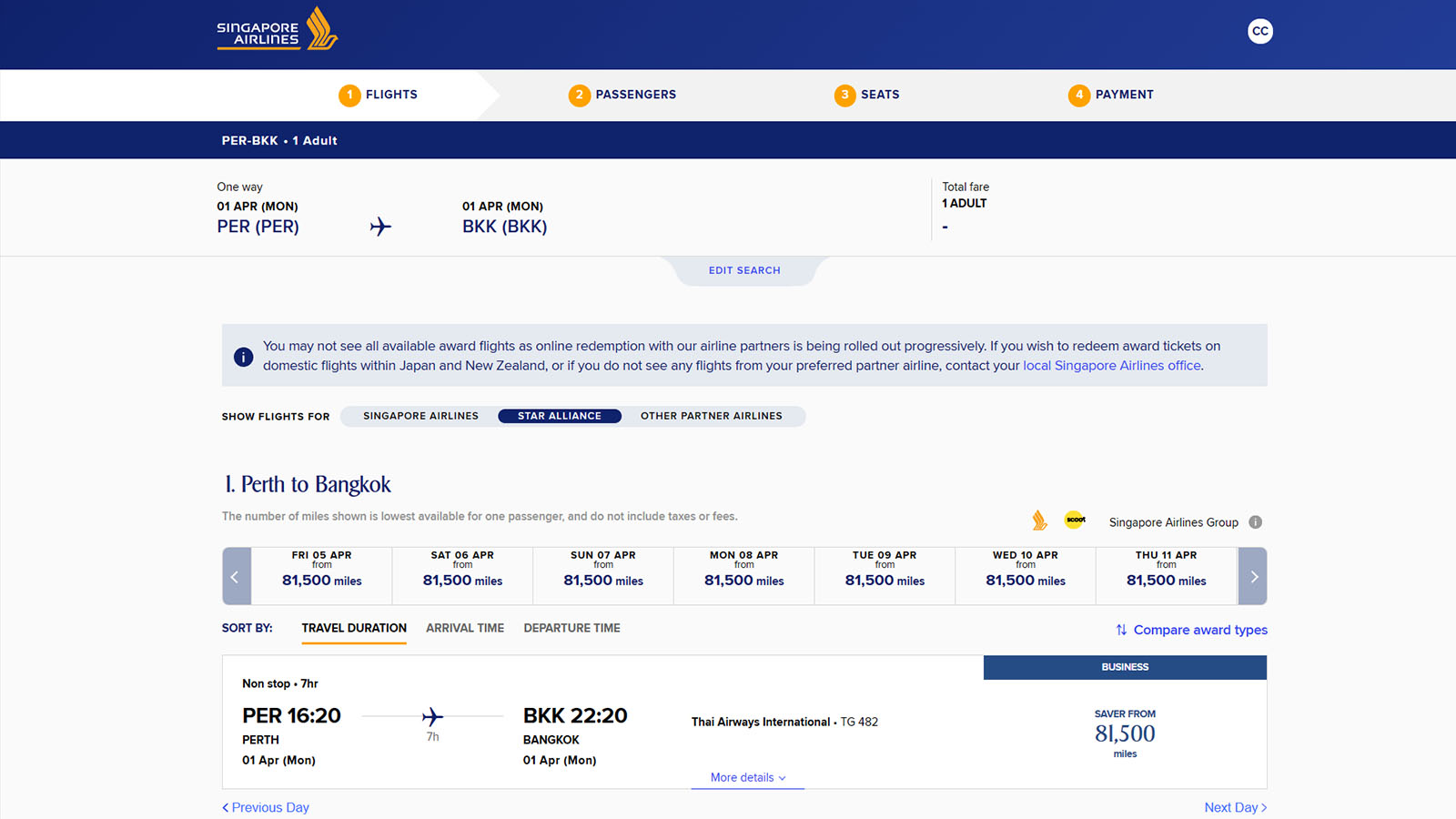**Caption:**

Screenshot of the Singapore Airlines booking webpage in landscape mode. The header features a blue stripe stretching from the upper left to the right-hand corner, showcasing the Singapore Airlines logo. Below, a white section displays a step-by-step process for booking a flight, with categories numbered in sequential order: 1. Flights, 2. Passengers, 3. Seats, 4. Payment.

A blue bar underneath indicates the flight details: "From BKK (Bangkok) to PER (Perth) for one adult, one-way on Monday, April 1st." Further down, an icon of an airplane signifies the flight date and type: "01 April, Monday - BKK to PER - Total fare for one adult." 

At the center, a section labeled "Edit Search" allows users to modify their flight criteria. A blue background below explains that not all available award flights may be visible online as the redemption system with airline partners is being progressively rolled out. For domestic flights within Japan and New Zealand or if preferred partner flights aren't displayed, travelers are advised to contact their local Singapore Airlines office.

Additional categories let users filter flights by Singapore Airlines, Star Alliance, or other partner airlines. The displayed itinerary shows a non-stop flight from Perth to Bangkok on Thai Airways International, taking approximately seven hours. The saver fare requires 81,500 miles, and several different dates are available for selection.